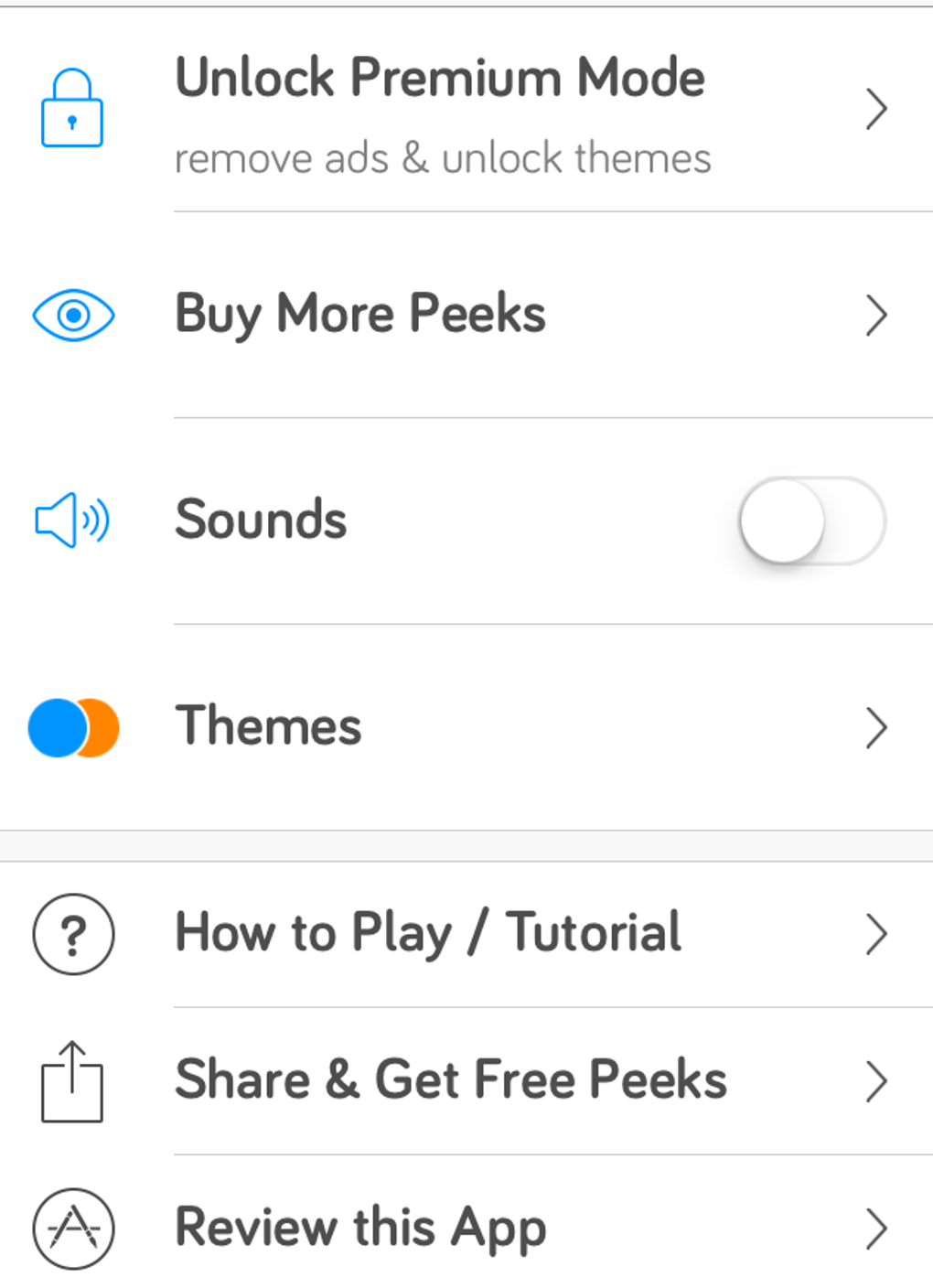This image depicts a mobile-friendly website interface with a series of options rendered in a highly readable format, characterized by large, bold, black text. The interface is bordered by a thick black line at the top, immediately followed by a prominent white bar. This white bar houses the text "Unlock Premium Mode" beside an icon of a blue lock to the left. Below this message, a subtitle reads "Remove ads and unlock themes," and to the right, there's a directional arrow pointing to the right.

Beneath the white bar, the next option is labeled "Buy More Peaks," in bold black text, accompanied by an icon of a blue eye on the left side and another arrow pointing right on the right.

Below this, the section labeled "Sounds" features an icon of a megaphone with emanating sound waves on the left. A slider switch icon to the right indicates the current state, which is off.

Following this is the "Themes" section, represented by intertwined orange and blue circles on the left, suggesting theme options, and another right-pointing arrow on the right.

A thin gray bar marks the boundary between sections. The subsequent section titled "How to Play Tutorial" includes a question mark inside a circle on the left and an arrow to the right.

Next, the option "Share and Get Free Perks" is illustrated with a sharing icon on the left, followed by another right-pointing arrow.

Finally, the "Review This App" option is marked with a circle containing an "A" to the left and the familiar right-pointing arrow to the right.